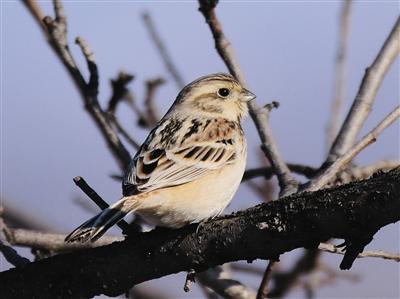In the photograph, a small, light-colored bird is perched on a thick, black branch. The bird, with a compact frame, features a cream-colored body accented by black and brown stripes on its wings and a black and white tail. Its head is marked with a dark stripe, and it has a small gray beak and beady black eyes. The bird is seen in profile, facing to the right. The background consists of a blurred mix of purple and blue-gray sky, complemented by scattered gray and brown tree branches shooting out from the trunk. The scene captures the bird calmly roosting, with intricate details of its plumage and the textured branch providing a striking contrast against the softly hued sky.